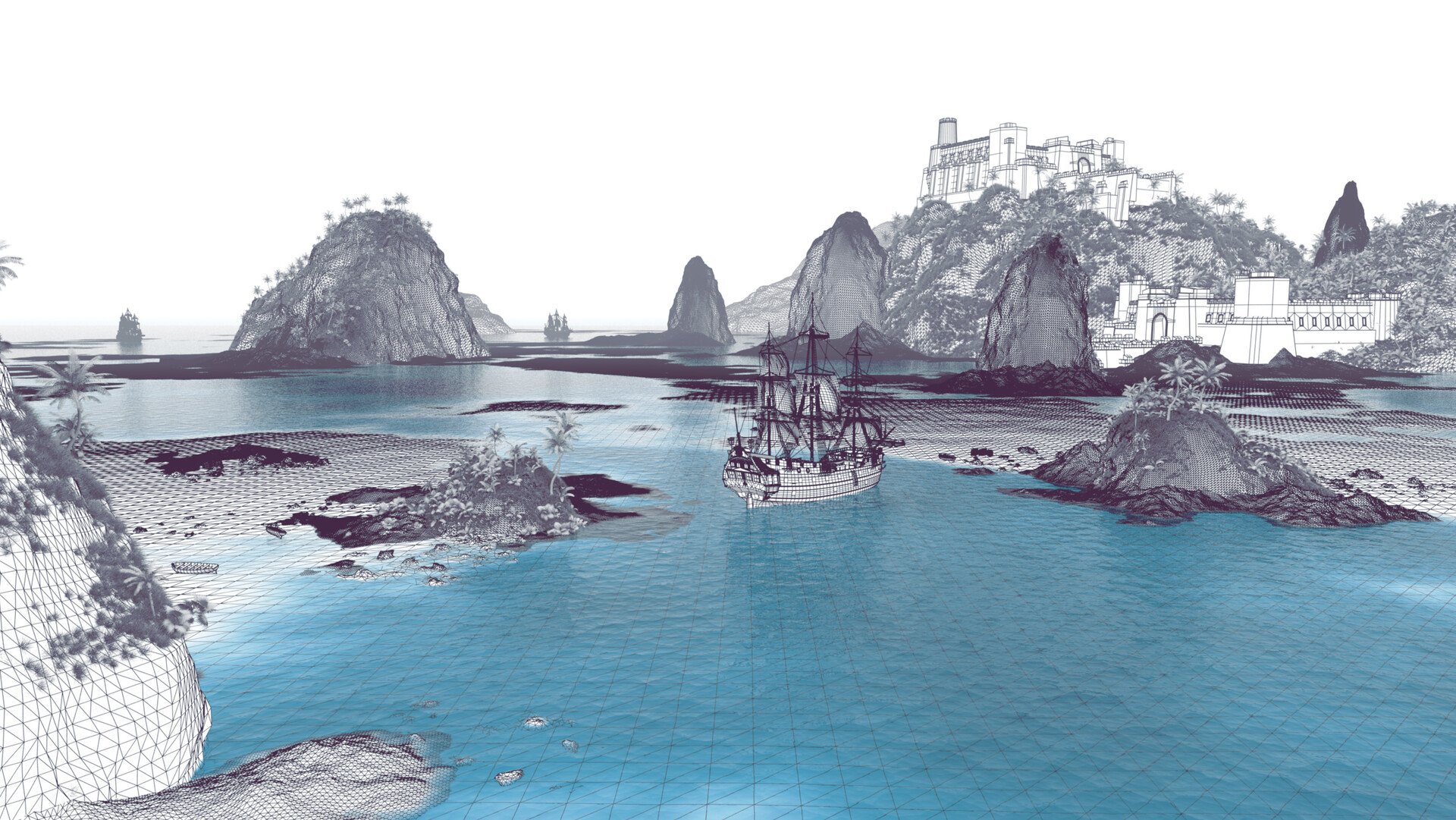In this outdoor scene, a bay with brilliantly blue water is dotted with large rock formations and small islands. A sailing ship, characterized by its black and white colors and lowered sails, sits amidst these rugged features. Along the serene shoreline stands a substantial white building, with another grand, white structure perched high on a hill behind it, which could be a house or a hotel. The sky above is a stark, plain white, contrasting with the detailed reflections of sunlight on the calm bay. Despite the expansive water, the exposed rocky terrain suggests the tide is out, creating a visually stunning, almost restrictive waterfront landscape.